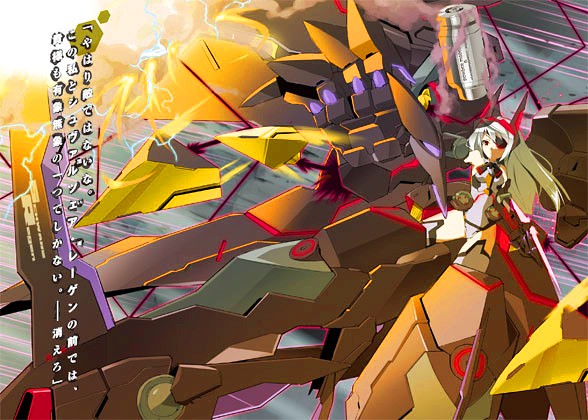The image is an intricate and animated piece of art featuring a symphony of vibrant colors, including yellows, blacks, browns, reds, blues, and grays, rendered in a variety of geometric patterns. The artwork appears to be an abstract and highly imaginative creation, possibly incorporating elements reminiscent of foam or cardboard cutouts with shapes in brown, orange, and yellow. Overlaying these cutouts is a complex scene dominated by Japanese characters written in three vertical rows on the left-hand side, and a central figure on the right-hand side.

The central figure seems to be a female character with whitish-blonde, long hair, partially morphed by a mechanical suit. This suit extrudes brown, robotic components resembling an oversized mechanical hand. The figure also features red ears protruding from her head and has one eye covered by an eye patch. The mechanical suit appears dynamic, possibly in mid-action, with yellow triangles emanating from it, suggesting a state of combat or engagement. The backdrop consists of a tablecloth with green and pink stripes, enhancing the overall collage-like aesthetic of the artwork, which blends traditional art forms with modern, animated elements.